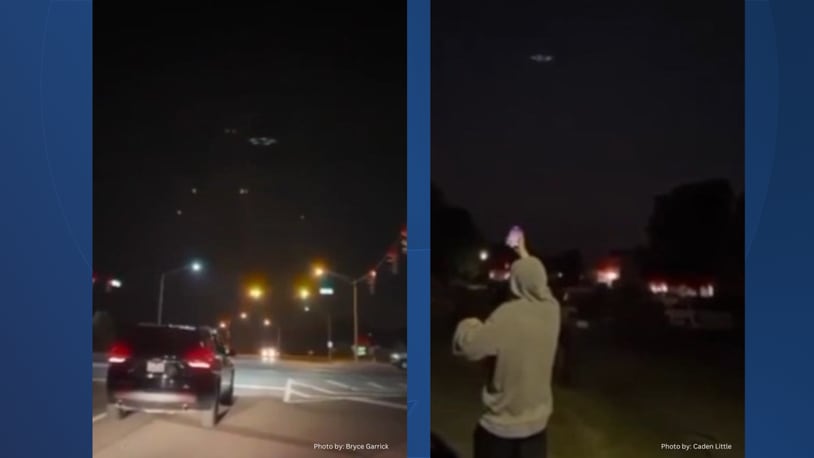The image consists of two separate nighttime photographs side-by-side, both capturing scenes from a city street. The left photograph showcases a dark SUV driving away under dim streetlights, with faintly visible white license plate and street markings, including a crossing area. The background is blurry, adding a mysterious ambience, and there is a notable UFO-shaped object in the sky. The bottom of this photo credits "Photo by Bryce Garrick." On the right side, the scene similarly unfolds during night-time in the city, featuring another dimly lit street environment. In the foreground stands a person in a khaki (or green) hoodie holding up a cell phone, seemingly recording or photographing the same UFO-shaped object seen in the left photo. This photograph is marked "Photo by Caden Little" at the bottom corner. Both images convey an eerie, captivating moment of urban life intersecting with a mysterious celestial phenomenon.